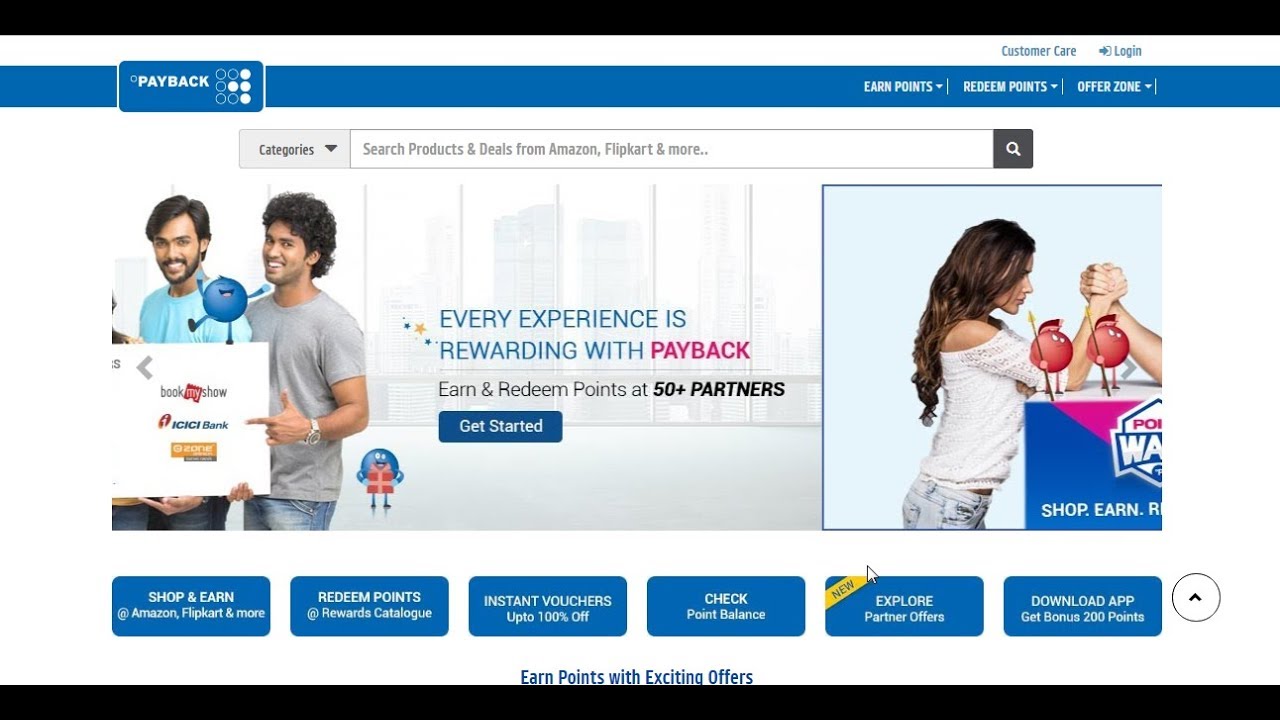Sure, here's a cleaned and detailed caption for the image:

---

The page, titled "Payback," features a cohesive and functional layout. In the top left corner, there's a small blue box with the word "Payback" written in white. Surrounding this are a series of dots, either blue with a white outline or completely white. Just to the right, there are three dropdown menus labeled "Earn Points," "Redeem Points," and "Offer Zone," each accompanied by a white downward arrow. Above these options, you’ll find "Customer Care" and a "Login" button.

Below this top section, the main content area includes a white search box prompting users to "Search Products and Deals from Amazon, Flipkart, and more." To its left is a dropdown menu labeled "Categories," while to the right, there's a grey search button highlighted with a magnifying glass icon.

To the left side of the main section, there's an image featuring two men holding a sign with a small blue character on top. The sign displays logos for "Book My Show," "ICICI Bank," and another entity labeled as "Zone." Adjacent to this image, a bold statement reads, "Every Experience is Rewarding with Payback. Earn and Redeem Points at 50-plus Partners. Get Started." On the right, there’s an image of a woman engaging in a friendly arm-wrestling match with an obscured person.

Beneath this main section, there are multiple blue buttons. The buttons read: "Shop and Earn" with mentions of Amazon and Flipkart, "Redeem Points," "Rewards Catalog," "Instant Vouchers up to 100% off," "Check Point Balance," "Explore Partner Offers," and "Download App Gift Bonus 200 points."

---

This caption maintains a comprehensive and detailed description of the page’s various elements.